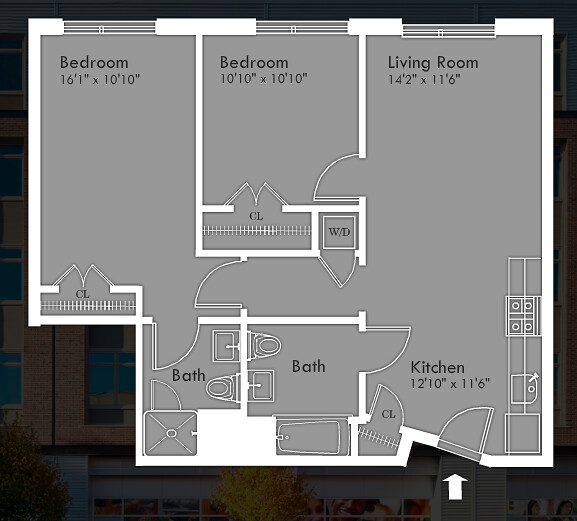The image features a detailed floor plan of a house, presented in grey with white outlines. The schematic layout highlights various living spaces including two bedrooms, a living room, two bathrooms, and a kitchen. Notably, one of the bedrooms contains an en-suite bathroom while the other does not. The floor plan specifies the dimensions for each room, excluding the bathrooms. Overlaying the floor plan is a faint, partially obscured image of a building in the background, adding a layer of context to the schematic but not detracting from the clarity of the layout.